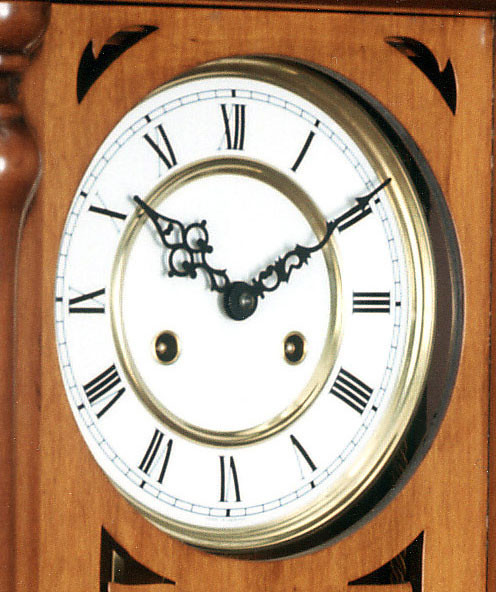This color photograph captures an up-close view of an old-fashioned grandfather clock. The clock is recessed inside a light brown wooden structure, which features intricate carvings allowing glimpses of its internal mechanism. The clock face is white, adorned with black Roman numerals from I to XII. Notably, the time displayed is approximately 10:10, with the black minute hand near the 9 and the hour hand pointing towards the 10. The clock hands have a unique design, almost resembling eyes. Encircling the clock face is a dual ring of gold, adding an elegant touch. Additionally, two small round gold circles with black interiors and gold dots are present. A slight brown pillar with two round spots is seen to the left, adding to the elaborate design of the wooden frame. The clock is protected by a glass covering, completing its vintage appearance.